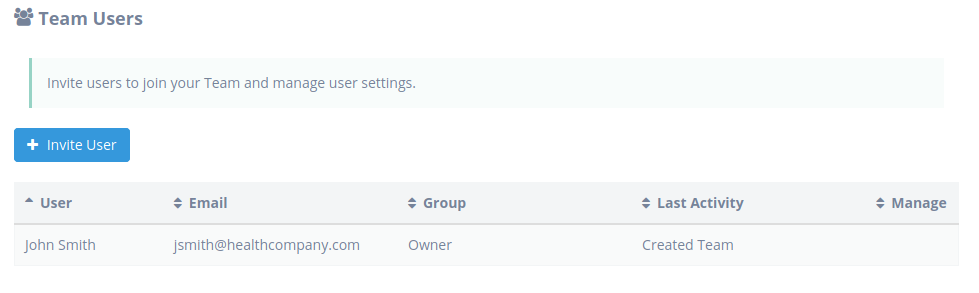In the left section of the image, there is a gray, almost flower-shaped icon with a distinctive design, where the top petal appears to be missing. This icon consists of a larger central circle surrounded by four smaller circles. Below this, there is a darker gray rectangle. Beside this icon, the words "Team Users" are displayed in gray letters. Underneath this text, there is a short vertical green line. Below that, a light-colored search bar area contains the text, "Invite users to join your team and manage user settings."

Further down, there is a blue rectangle featuring a white plus sign inside, labeled "Invite User." Below this button, there is another long light gray rectangle divided into several columns. The column headers read: "User," "Email," "Group," "Last Activity," and "Manage."

Under the "User" column, the entry reads "John Smith." In the "Email" column, the entry is "jsmith@healthcompany.com." The "Group" column indicates "Owner." The "Last Activity" column shows "Created Team." The "Manage" column is empty.